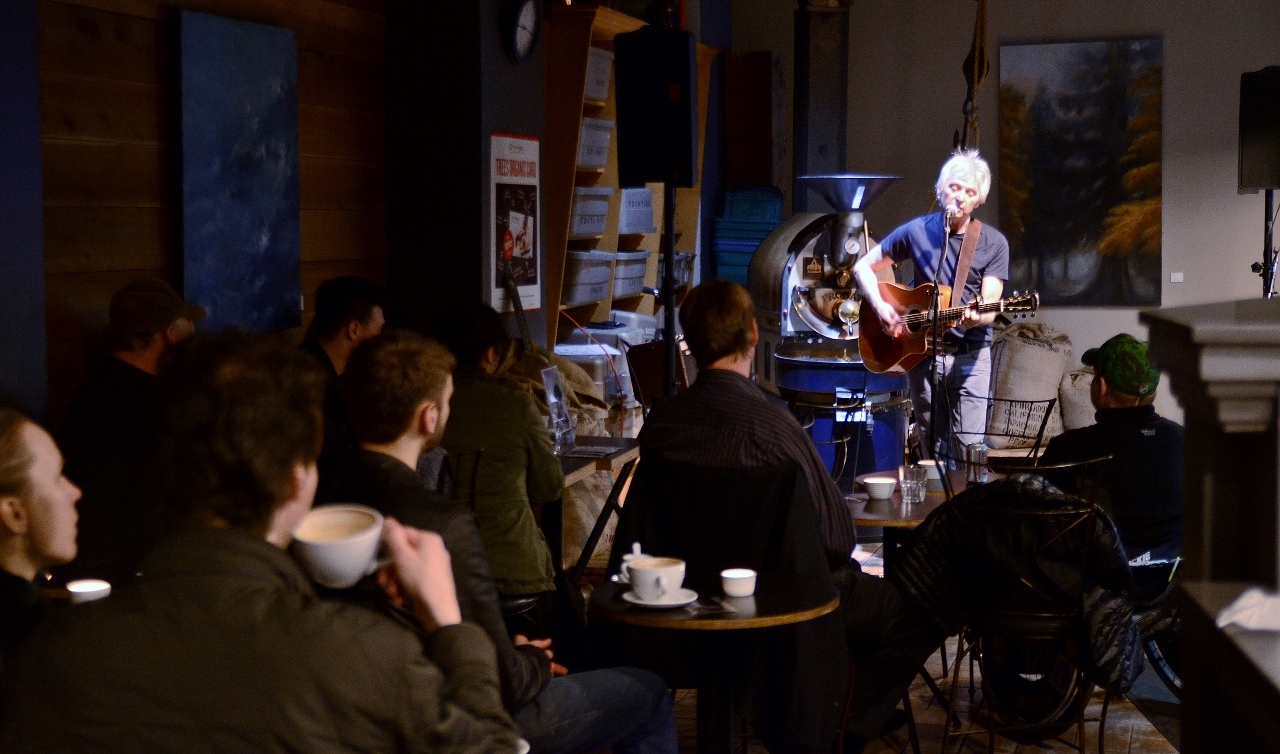In this photograph taken from the back of a cozy coffee shop, a crowd of young male patrons is seated at tables, sipping on their coffee or lattes, and focusing intently on a performer at the front. The performer, an older man in a blue short-sleeved shirt with white hair, is playing an acoustic guitar, entertaining the audience as they enjoy their beverages. The setting appears warm and inviting, with elements like a possible coffee bean grinder, nature-themed paintings, and lamps adding to the ambiance. The lack of text in the image allows the details and colors—ranging from white and dark blue to shades of brown and a hint of red—to speak for themselves, suggesting a serene, indoor venue that could either be day or night. The scene captures a moment of live music in a typical coffee shop atmosphere, where products may also be displayed for sale.